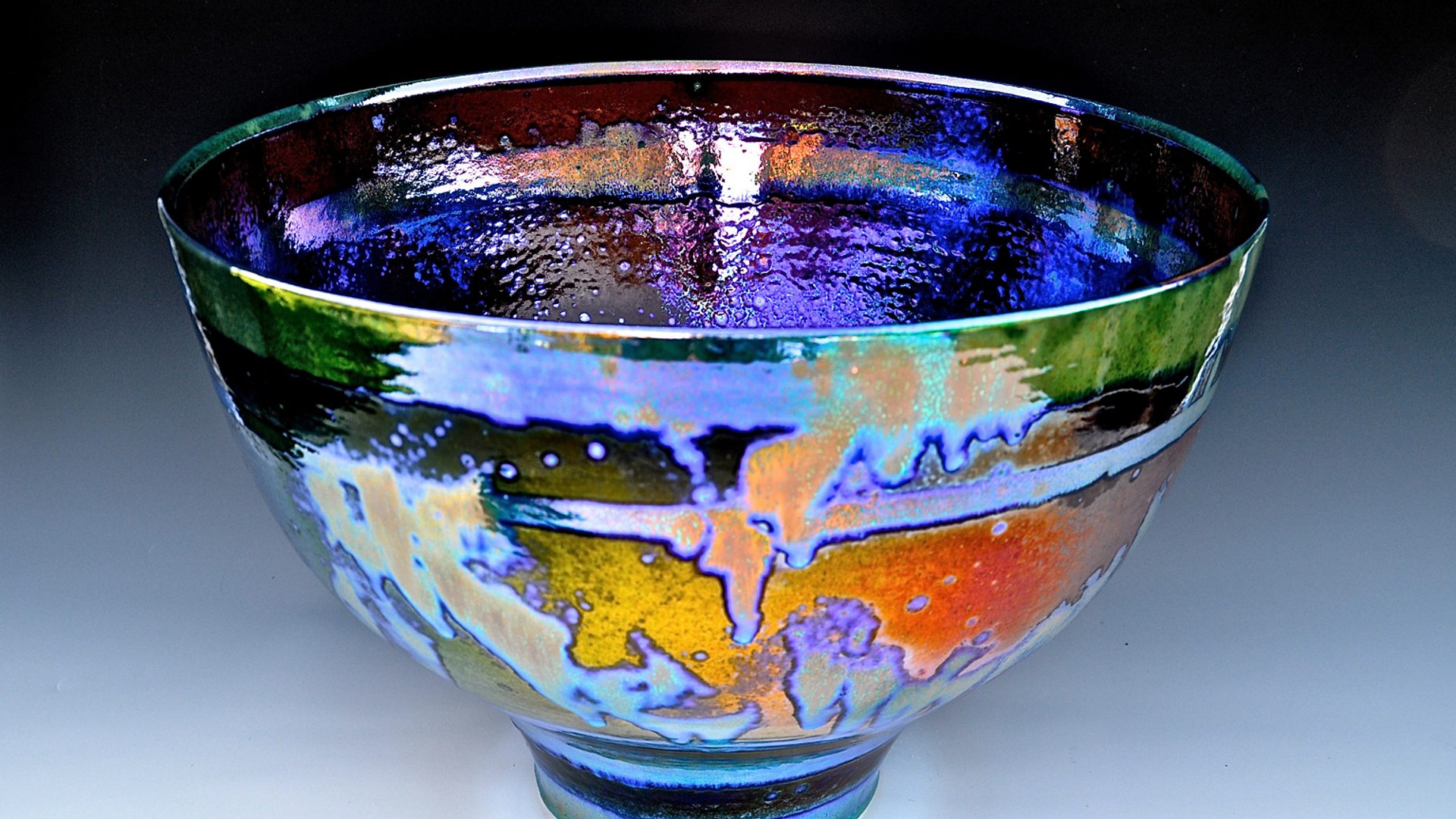The image captures a close-up of an extraordinarily unique footed bowl that appears to be crafted from either glass or a metallic material, giving it a stunning iridescent sheen. The bowl is round, deep, and features a mesmerizing array of colors that shift when viewed from different angles, including green, orange, blue, white, purple, and a hint of crimson red. The bowl is perched on a base approximately 1-1.5 inches high, adorned with detailed blue and silver bands that encircle it. The exterior of the bowl exhibits an abstract, splotched appearance—colors like green, silver, yellow, and orange appear to run and blend together, creating dynamic outlines where the silvers meet other hues. The inside of the bowl glows with iridescent purple and blue tones, reflecting light in a way that adds depth to its dark interior. The entire composition sits against a background that fades vertically from light gray at the bottom to a near-black at the top, emphasizing the bowl's vibrant and ever-changing color palette.